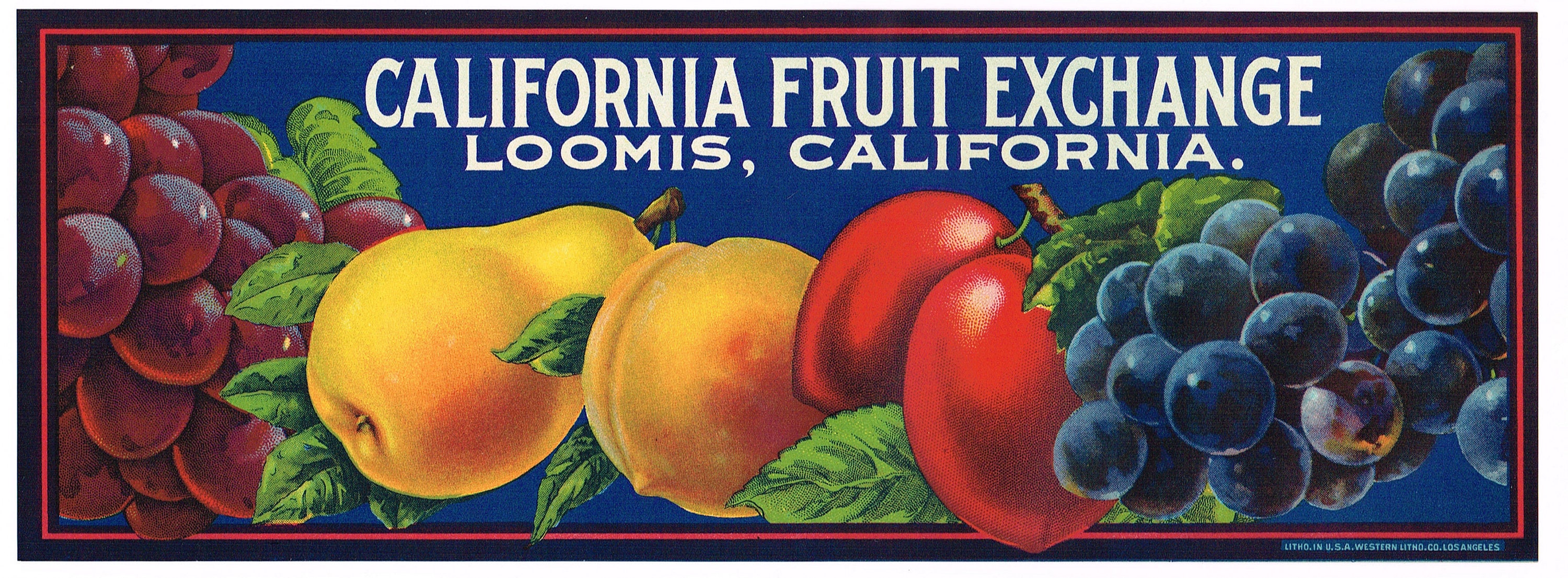This vibrant, rectangular advertisement poster features a rich blue background framed by a thin red pinstripe and a bold black border. At the top, in striking white text, it reads "California Fruit Exchange, Loomis, California." Below this title, a beautifully detailed collection of painted fruits is showcased. To the left, clusters of red and purple grapes adorned with green leaves catch the eye. Adjacent to these grapes sits a bright yellow pear with a small branch protruding from its top, surrounded by more green foliage. Next comes an orange-hued peach, followed by two red fruits, likely tomatoes, depicted with one in front of the other on small branches. Finally, towards the far right, a cluster of blue grapes completes the arrangement. The overall composition is a harmonious blend of colors and shapes, with leaves interspersed throughout, enhancing the natural beauty of the depicted fruits. At the bottom right, there is a faintly legible signature, and inscribed in bluish text along the black outline, it reads "Litho in USA, Western Litho Co Los Angeles."